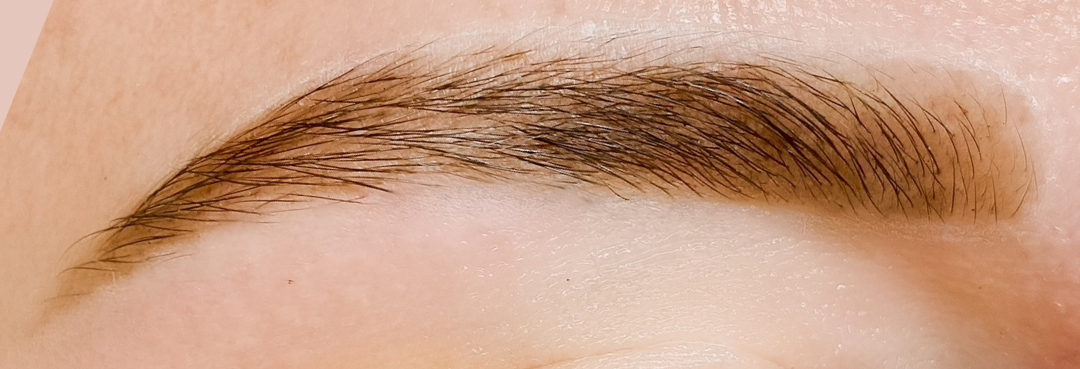This close-up image captures a finely tweezed right eyebrow with brown hair set against smooth, ivory skin. The detailed focus reveals the natural arch of the brow just above the eyelid and a very small mole underneath on the left side of the image. The skin appears smooth with some pores visible but nothing unnatural. The background includes a hint of pink in the upper left corner. The photograph, presented in a horizontal rectangular format, likely serves a beauty-centric purpose, possibly related to eyebrow waxing or makeup. The clean and detailed close-up shows the intricacies of the well-groomed eyebrow and the subtly tinted skin beneath.